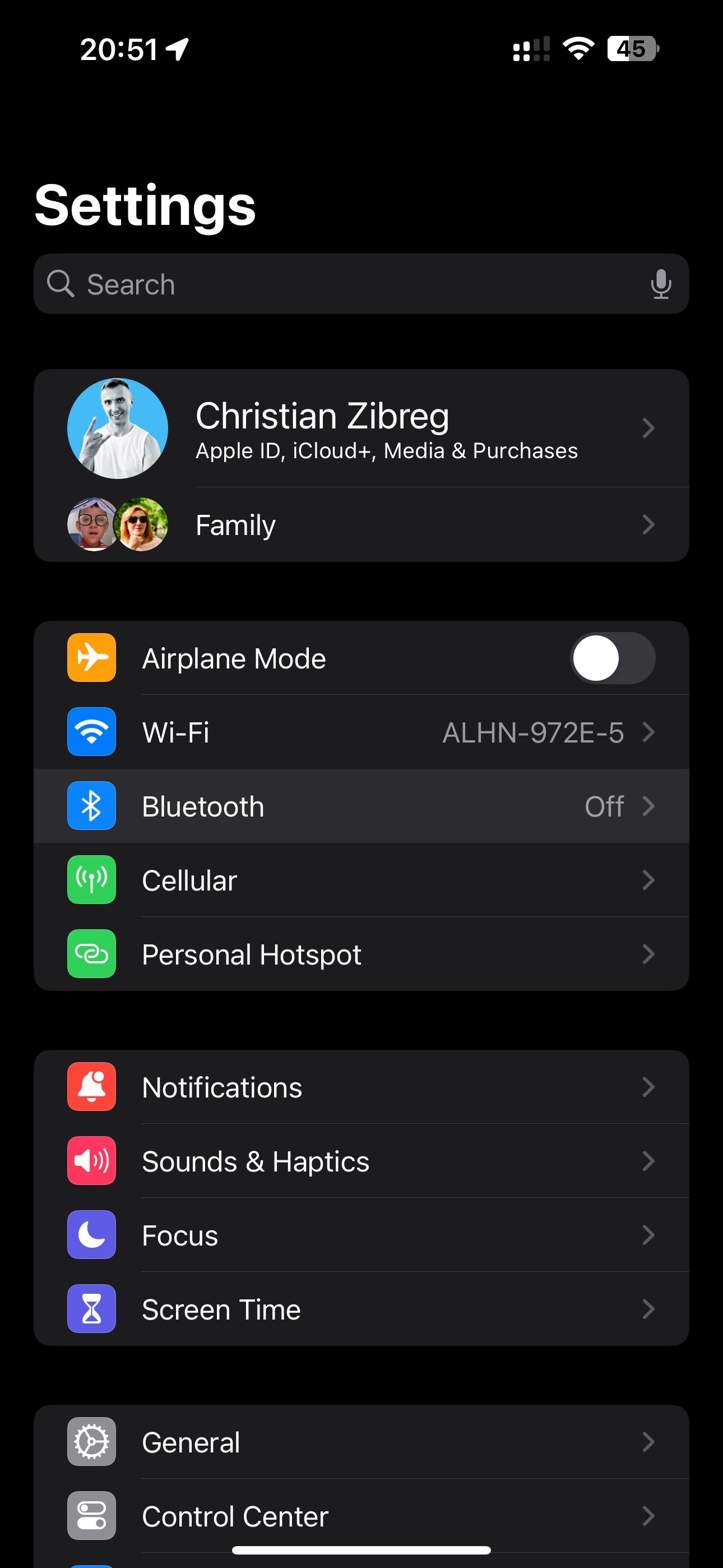In the image, a smartphone screen displays the settings page against a completely black background, with all text in white. The top section starts with a search bar labeled "Search," followed by a section dedicated to the Apple ID, showing the name "Christian Zbreg" and sub-options for "Apple ID," "iCloud Plus," and "Media Plus Purchases." An icon representing Christian Zbreg, with a light blue background, features a male figure. Below this, the "Family" section shows two icons depicting what seem to be female figures. The settings include several options listed in gray sections: "Airplane Mode," which is toggled off; "Wi-Fi" connected to network "ALHN-972Z-5"; "Bluetooth," which is off; "Cellular;" "Personal Hotspot;" then "Notifications," "Sounds & Haptics," "Focus," and "Screen Time." Further down, options for "General" and "Control Center" are also visible. The time at the top left of the screen reads 20:51. The top right corner shows symbols indicating active Wi-Fi and a battery at 45% charge. Overall, the image captures a comprehensive overview of a cell phone's settings page.